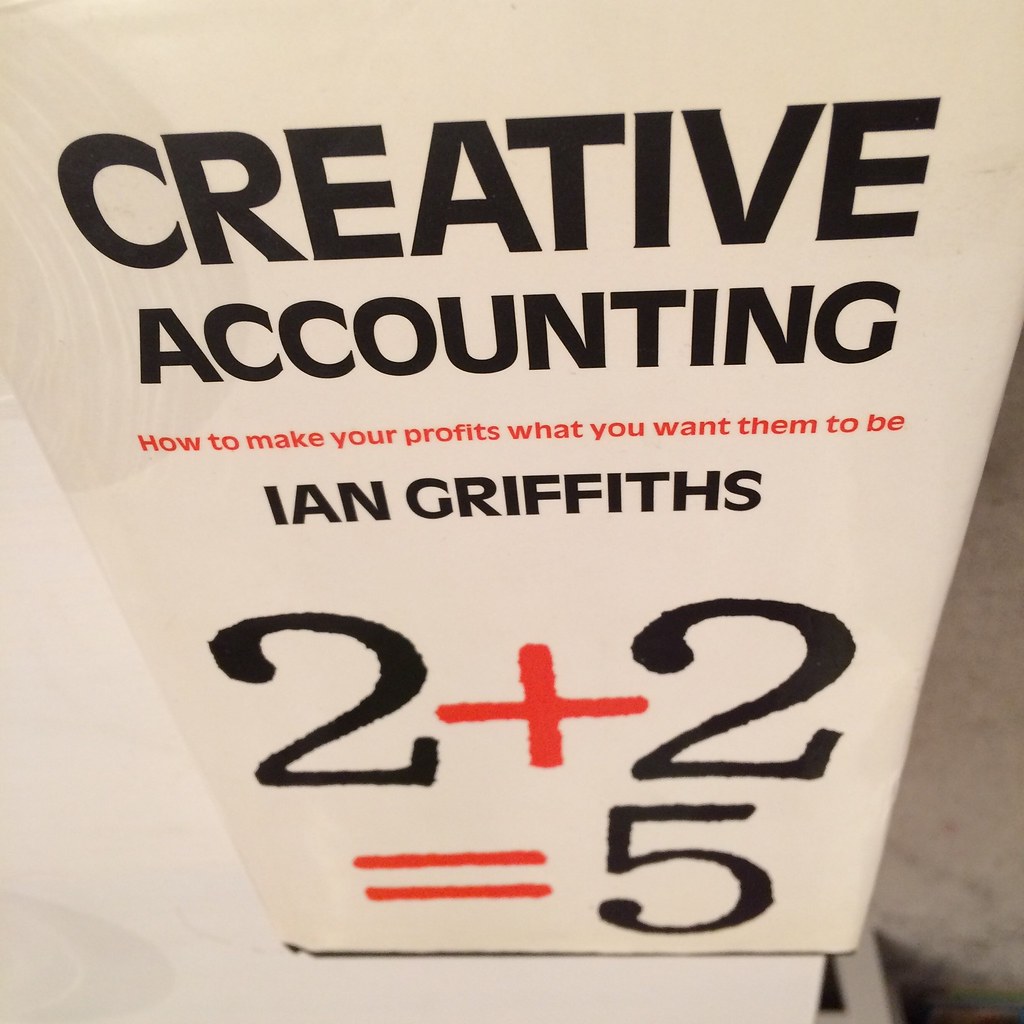The image features a close-up photograph of a book with a white and black cover, resting on an off-white, beige surface. The cover has a shiny coating that reflects light and surrounding objects. The title "Creative Accounting" is prominently displayed in bold black text across the top. Below the title, a subheading in smaller red text reads, "How to make your profits what you want them to be." Beneath this, in black text, is the author's name, Ian Griffiths. At the bottom, there is an equation: "2 + 2 = 5," where the numbers (2s and 5) are in black and the plus and equal signs are in red. The background of the photograph varies in tones of gray and beige, giving a somewhat off-white, creamy appearance.